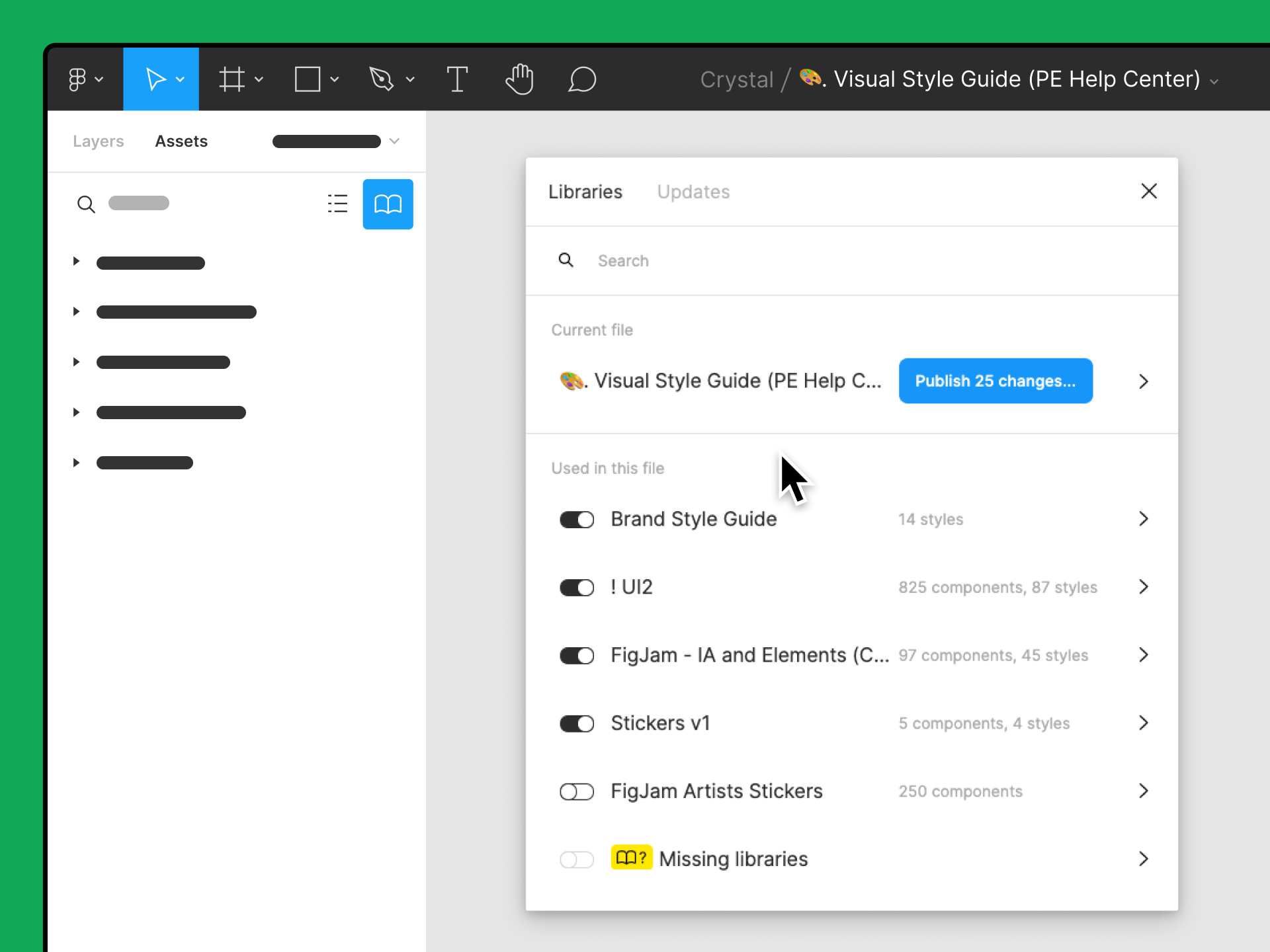This image appears to be a detailed screenshot of a web application mock-up or design prototype, featuring a comprehensive user interface.

The borders on the left and top sides are highlighted in green. The top border includes a series of distinctive icons: an 'F', an arrow, a tic-tac-toe grid, a square, a pen, the letter 'T', a hand, and a word bubble. Positioned next to these icons, the word "Crystal" is displayed, followed by an icon representing a paint set. Adjacent to these elements, the text "Visual Style Guide PE Help Center" is visible.

On the left side below the top border, there is a vertical white column labeled "Layers" and "Assets." This column includes a series of gray bars, presumably placeholders for text. It also features a search field, a book icon, and a hamburger menu icon.

To the right of this column is another white box labeled "Libraries." This section contains various options for different style guides, each accompanied by slider controls that are either turned on or off, along with additional descriptive information.

Dominating the center of the screen is a large cursor icon, which is black with a white outline and a slight drop shadow, underscoring its prominent placement in the mock-up.

Overall, this image seems to represent a detailed design prototype of a web application, rather than a functioning application.